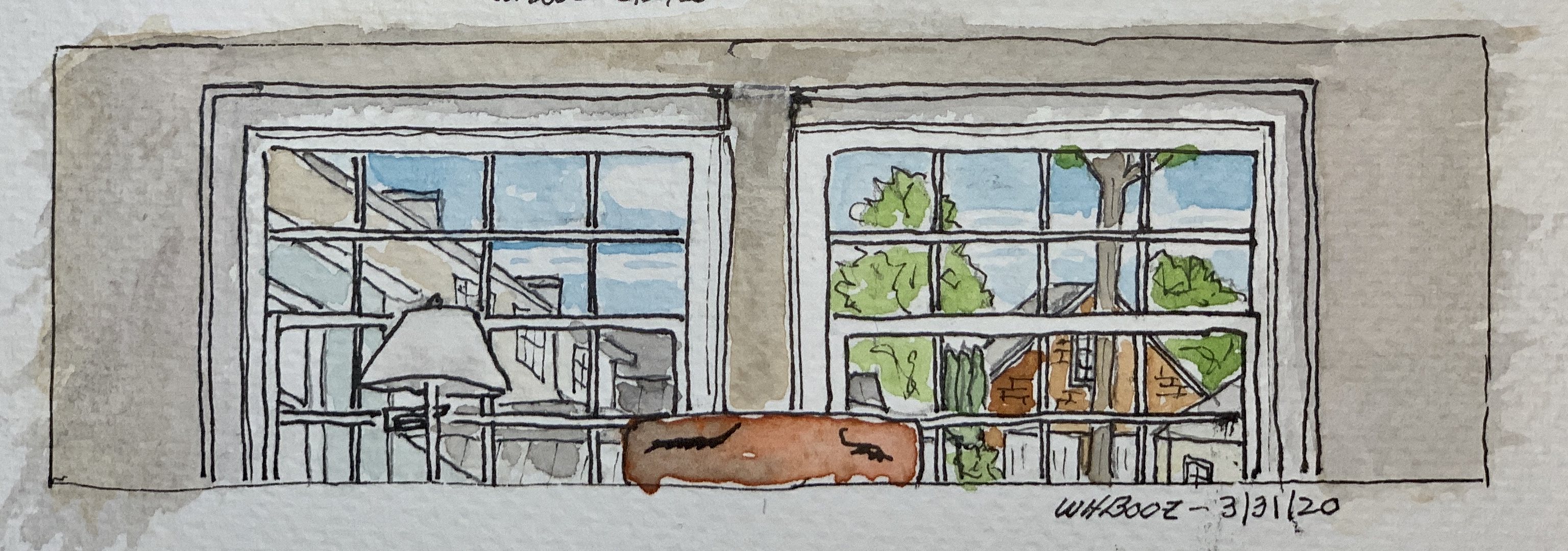This is a detailed watercolor painting resembling a comic book strip, signed "W. H. Booze-33120" at the bottom right. The image predominantly features two white-rimmed windows, through which viewers can see an outdoor scene. The exterior showcases a mix of buildings, including a two-story commercial or apartment building that is partially brown and white, and a residential home constructed of brown stone with a triangular roof. Several trees punctuate the view, and the sky above is blue with scattered clouds. Inside the room, in front of the windows, there is a tall white lamp and a brown chair positioned against a tan-colored background. The painting is set within a gray border that has a subtle brown overlay, adding depth to the image. The overall effect is reminiscent of a carefully rendered sketch, with a detailed and nostalgic quality.